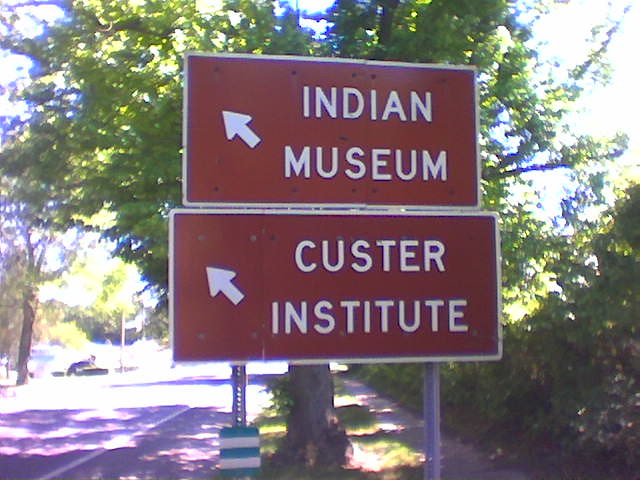The image depicts two U.S. National Parks road signs situated on the side of a gray paved road, which features a white line running along its edge. The road is bordered by a patch of green grass with a tree, whose dark green leaves show lighter shades where the sunlight hits them. Adjacent to the grass is a thin gray sidewalk. The signs are mounted on two metal posts with slots in them. The upper sign reads "Indian Museum" with a white arrow pointing to the northwest. The lower sign directs to "Custer Institute," also with a white arrow pointing to the northwest. Both signs have a maroon background with white text and are outlined in white. A small green and white square sign is placed in front of the posts. Additionally, there are some shrubs and another tree visible in the grassy area. The scene is bathed in bright sunlight, suggesting a clear, sunny day.